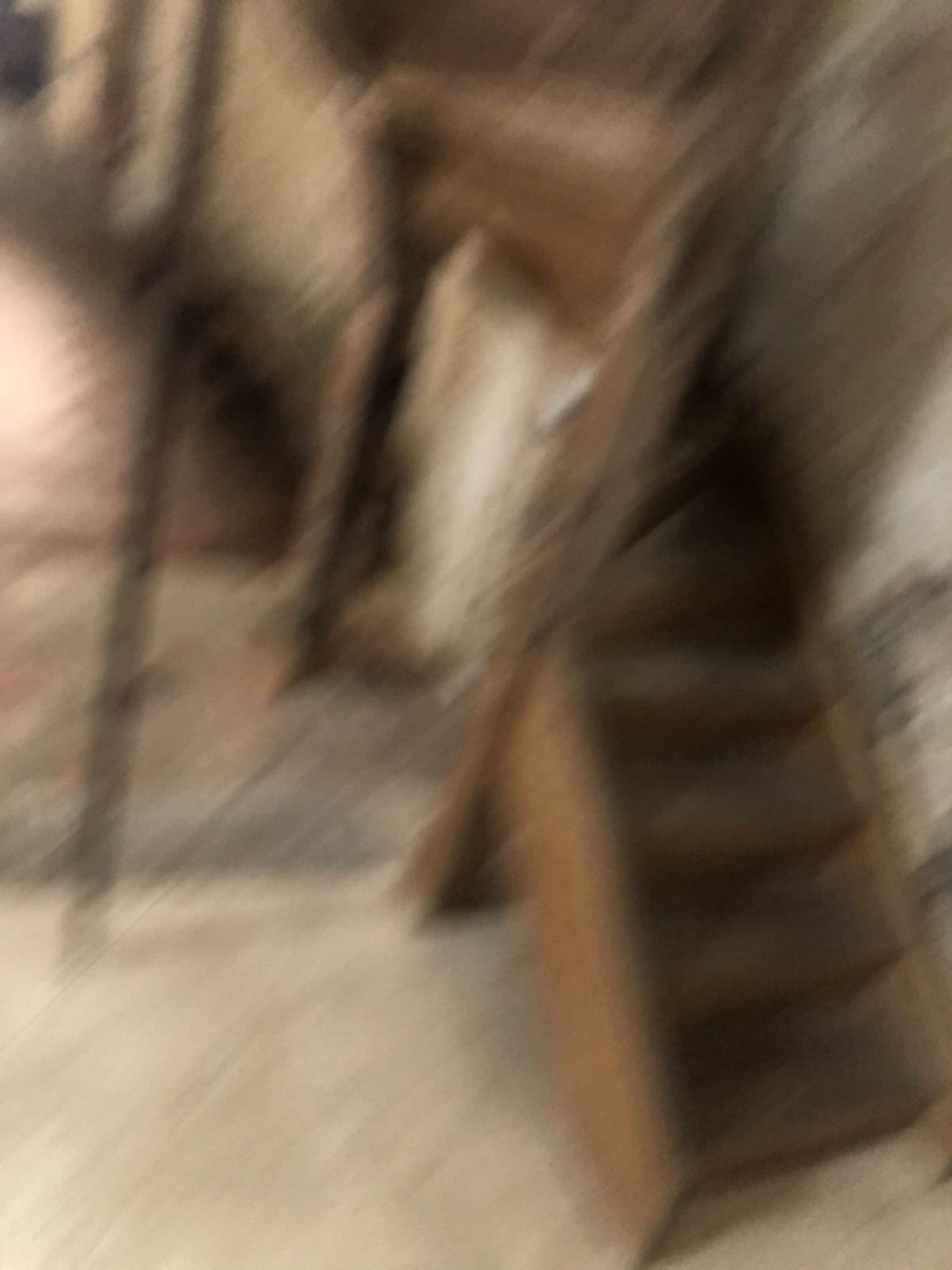A heavily blurred photograph showcasing a set of wooden stairs occupies the right-hand side of the image. The stairs, composed of beige-brown wood, appear to wind slightly at the top, though only the lower sections are clearly discernible. A light beige-white floor contrasts subtly with the stairs, leading to a similarly hued wall in the background. The overall effect is marred by significant blurriness and streaks, giving the impression of motion or a shaky camera, most likely taken with a smartphone.